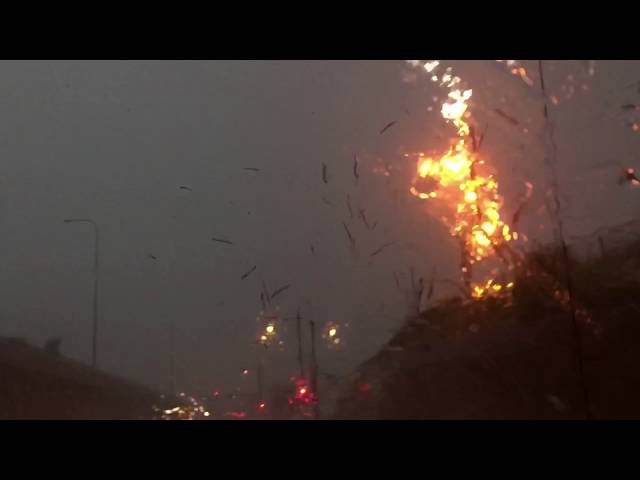In this stark nighttime photograph, there is a dramatic scene of an intense blaze consuming a hilltop in a semi-urban area. The dark sky is illuminated by the bright yellow and orange flames shooting up from the hill on the right side of the image. Bits of burning debris, possibly shrubbery or connected material, are flying through the air. The viewer's vantage point seems to be from a car, looking up at the fiery scene. Tall street lamps and lampposts line the road, illuminating the otherwise dark surroundings. The lights from distant structures and streetlights suggest this might be a drizzly evening, at dusk or nightfall. The photograph does not depict any people or animals, focusing solely on the intense fire and the scattered remains of what could be wood or metal fragments, adding to the sense of chaos.